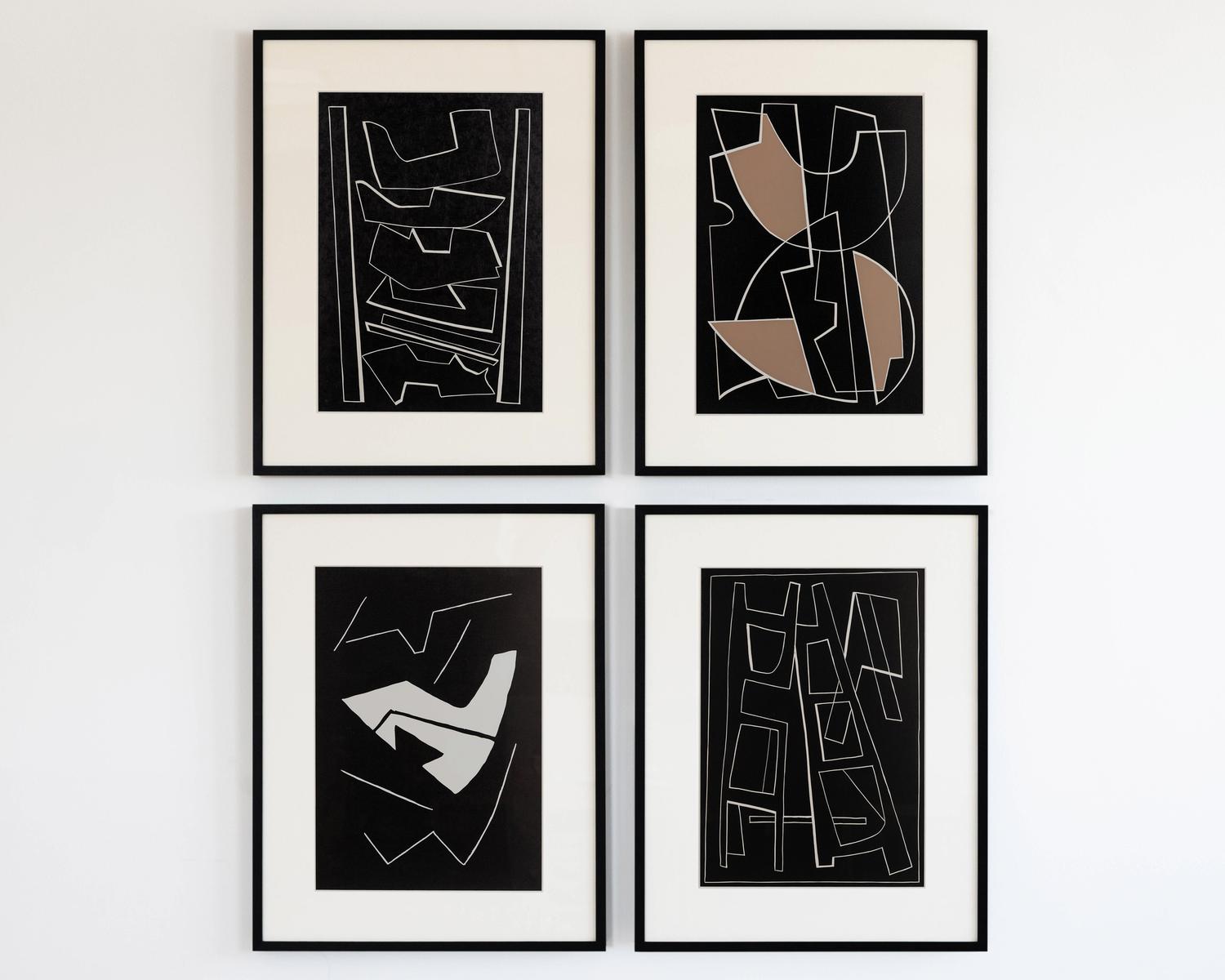The image features four vertically rectangular framed artworks evenly spaced on a white wall, arranged in a square formation with two on the top row and two on the bottom. Each artwork is framed in a black border with a white mat surrounding the abstract pieces, all containing black backgrounds accented with white and tan geometric shapes.

The top left artwork showcases a series of six stacked brackets pointing upwards, flanked by two vertical straight lines. The top right piece is characterized by an array of rectangles and half-circles, incorporating a mix of black, white, and tan elements. The bottom left frame presents representations reminiscent of a mouth, nose, and chin, depicted through abstract white lines and shapes such as a butt chin, a jagged mouth, and a triangular nose. Finally, the bottom right artwork features white line designs resembling two parallel ladders alongside a structure suggestive of a step ladder, contributing to the cohesive yet unique abstract theme shared amongst all the pieces.